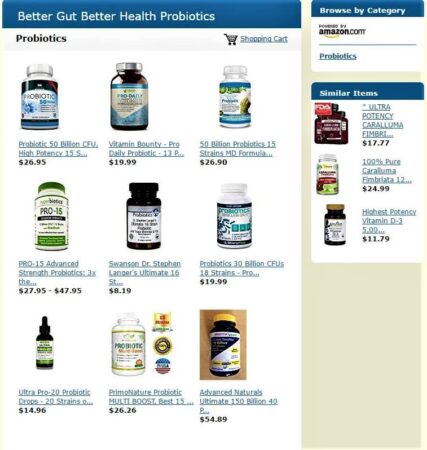The image features a detailed layout of a webpage segment focused on probiotics. On the left side, there is a dark blue header with slightly fuzzy white text that reads "Better Gut, Better Health Probiotics," indicating low image quality. Below this header, in black text, the word "Probiotics" is displayed. To the right of this section, there is a black shopping cart icon with a blue, underlined label "Shopping Cart," signifying a clickable URL.

Further to the right, a rectangular area with a dark blue header background prominently displays the bold white text "Browse by Category." Beneath this header, the Amazon.com logo appears, with "Amazon" in bold black and ".com" in a thinner black font. Below the logo, there is a gray-bordered section featuring an underlined, blue text link that says "Probiotics."

Directly beneath, there is an elongated rectangular area with rounded corners. The top part of this area also has a dark blue header with bold white text that reads "Similar Items." Below this header, three different supplement names are listed along with their prices. The first product, "Ultra Potency C-A-R-A-L-L-U-M-A F-I-M-B-R-I..." is priced at $17.77 in black text. The second item features an image of a bottle with a green lower section and a red oval, labeled "100% Pure C-A-R-A-L-L-U-M-A F-I-M-B-R-I-A-T-A 12...," with a bold black price of $24.99.